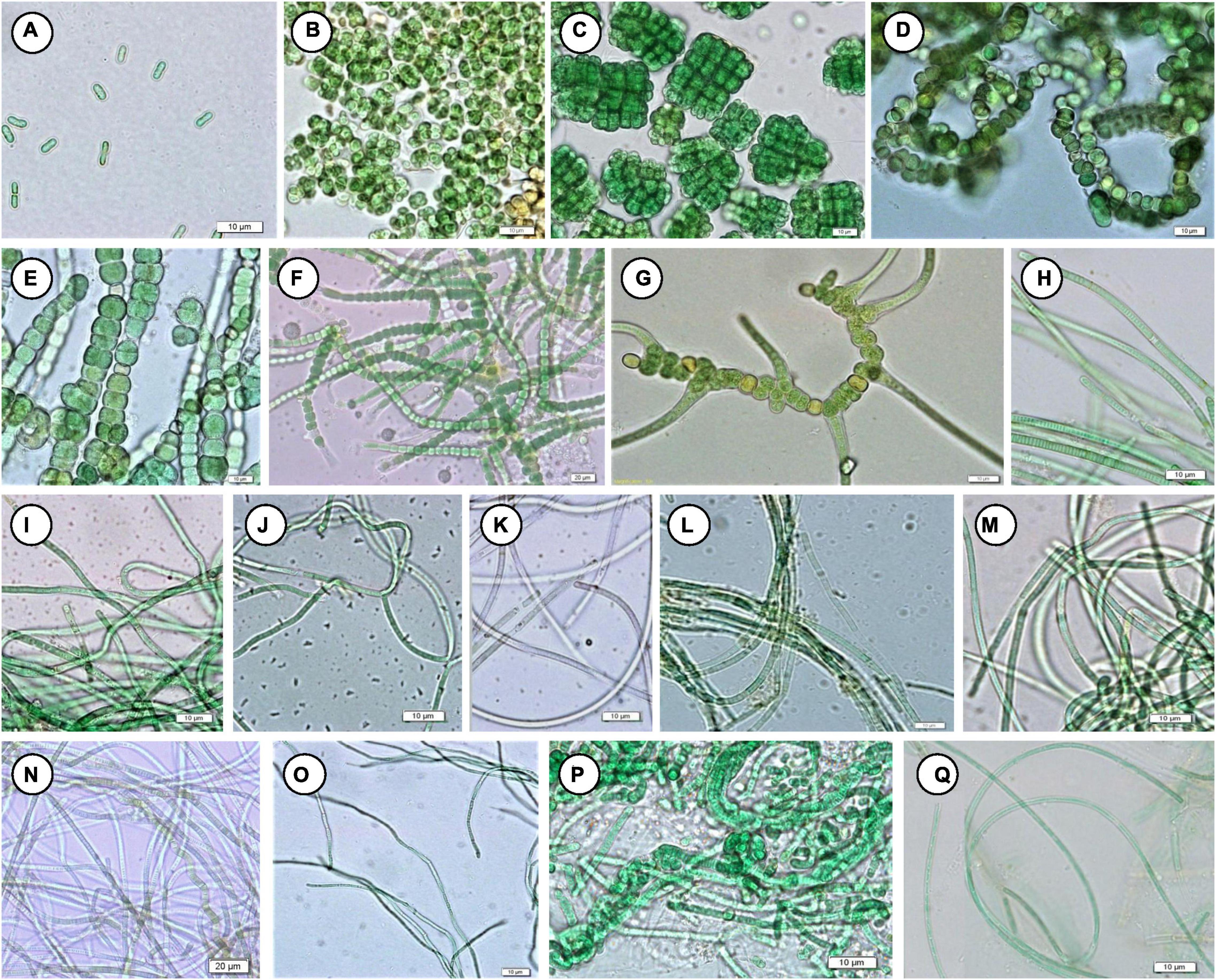The image is a detailed array of 17 labeled photographs taken under a microscope, showcasing various microorganisms, potentially algae or bacteria. The photographs are arranged in four rows, labeled from A to Q. The first row features images A, B, C, and D; the second row includes E, F, G, and H; the third row has I, J, K, L, and M; and the fourth row contains N, O, P, and Q. Each image displays a pale gray or bluish background with green organisms of different shapes and sizes. Some organisms appear as long, slender chains, resembling glass, while others are cube-like or bead-like in structure. Each photograph also includes a scale in the bottom right corner, likely in micrometers, though it is difficult to read. Overall, this collection of microscopic photographs offers a fascinating glimpse into the diverse morphology of microscopic life forms.